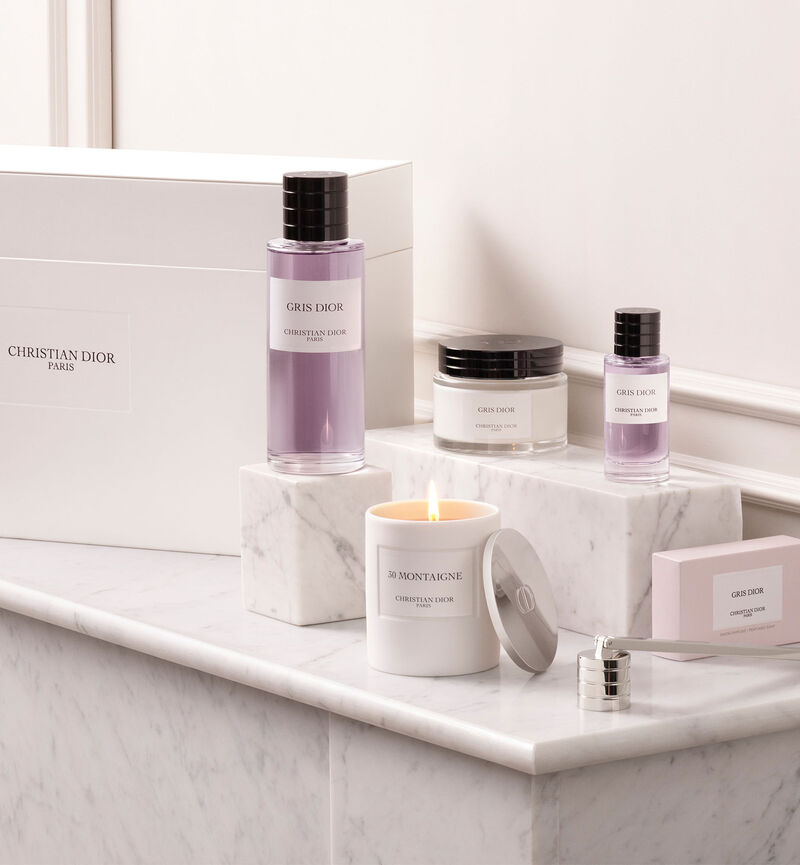This image features an elegant product placement for the luxury brand Christian Dior. Displayed prominently on marble blocks and a marble countertop, the arrangement includes a variety of items, making it a sophisticated set likely intended for gifting. At the center of the display is a lit white candle with a yellow flame, bearing the label "30 Montaigne, Christian Dior Paris," and a silver pop-off lid. To its right is a box of soap in a pink container, also adorned with the Christian Dior label.

A clear glass bottle containing a pink liquid sits nearby, with the label "Gris Dior, Christian Dior Paris" in black serif font, featuring a sleek black cap. A smaller travel-sized version of this bottle implies it could be perfume or cologne. Additionally, there's a clear plastic jar of cream, with a matching label and black lid, positioned towards the back.

Completing the ensemble, a stylish white rectangular gift box with "Christian Dior Paris" printed in black letters is placed on the left. This gift packaging, along with all the products, is set against a white wall accented with crown molding. A metallic-colored candle snuffer with a handle can also be spotted, perhaps to put out the candle safely, enhancing the luxurious and practical nature of the collection.